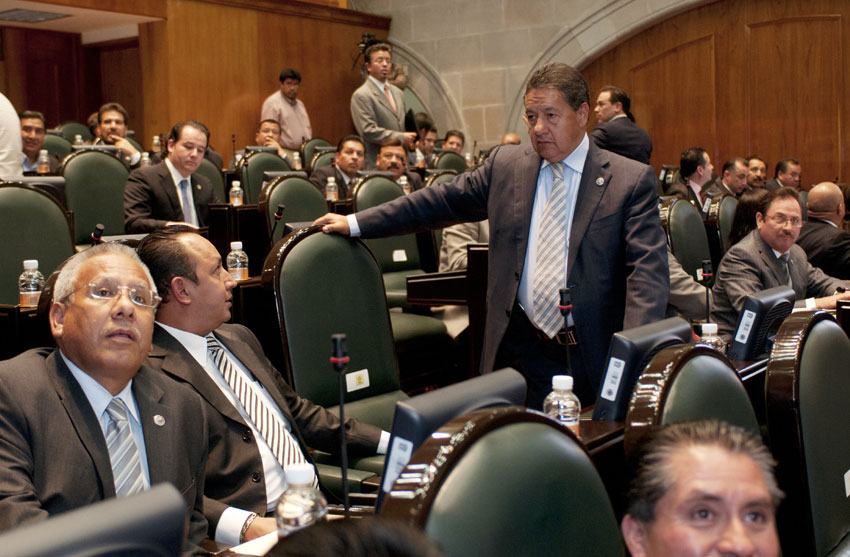This full-color photograph, taken indoors, captures an important meeting with an all-male audience. The room features brown paneled walls interspersed with sections of stone wall made from concrete blocks, as well as a decorative granite archway. The attendees are seated in elegant green leather chairs behind dark brown desks, each equipped with a monitor screen, console, or computer, and a microphone. Bottles of water are positioned in front of each person. Most gentlemen are wearing suits and ties, with the exception of one man in the far back wearing just a shirt. Central to the image is a man in a dark blue suit standing and facing left, engaged in conversation with a seated man in a suit and brown-striped tie. Some attendees are looking towards the stage at the far left or a screen in the upper right of the photograph, suggesting presentations or discussions are taking place.